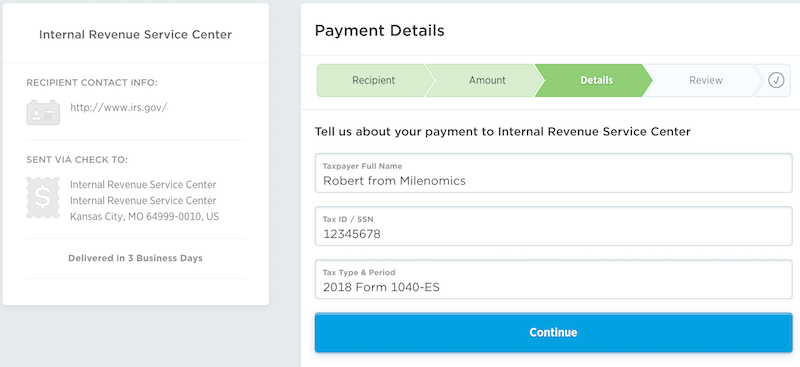This screenshot captures a detailed view from the IRS website, specifically the Internal Revenue Service Center's payment section. The page is divided into two main sections. On the left, it shows the recipient contact information: payment to be sent via check to the Internal Revenue Service Center in Kansas City, Missouri, with an estimated delivery time of three business days. The web address provided is www.irs.gov.

On the right side of the screen, the payment details are visible. A progress bar at the top indicates the current phase of the transaction, which includes steps labeled as recipient, amount, details, review, and confirmation (check mark). The screenshot is in the 'details' phase of this sequence. 

The section is titled "Tell us about your payment to Internal Revenue Service Center." The form fields indicate that the taxpayer's full name is Robert from Milonomics with the Social Security Number 123-45-6789. The tax type and period specified are for the 2018 Form 1040-ES. A blue 'Continue' button is highlighted at the bottom of the form.

The overall context suggests that this screenshot guides users through a process of making a payment, possibly for back taxes, with a clear status tracker showing the user is in the details phase of their payment submission.